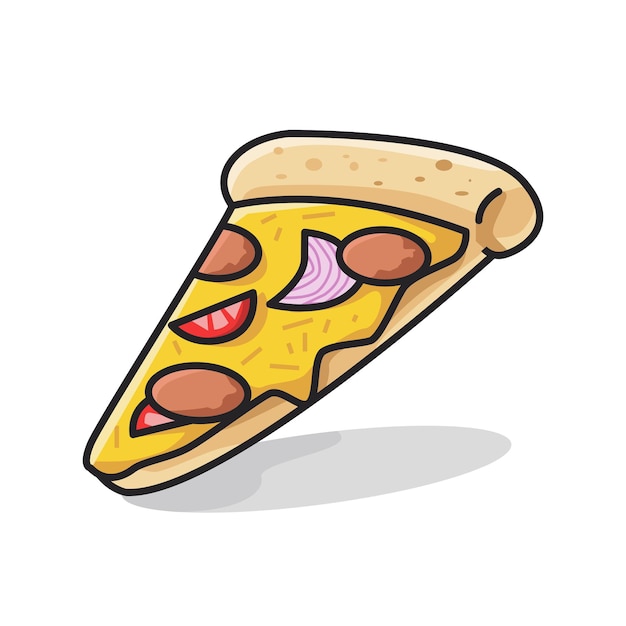This image depicts a simple, cartoonish drawing of a slice of pizza against a white background. The slice is propped up, resting on its triangular tip with the rest floating slightly above, casting a circular blueish-grey shadow below. The pizza features a light brown crust with darker brown spots, outlined thickly in black, enhancing the cartoony, clip-art style. The cheese, a mustard-like golden yellow, covers the slice, topped with three brown circles resembling pepperoni. Additionally, there are two small red half-circles, likely tomatoes, and a white, 3/4 circle with purple stripes, possibly representing an onion. The overall illustration is simple and playful, reminiscent of a comic book aesthetic.